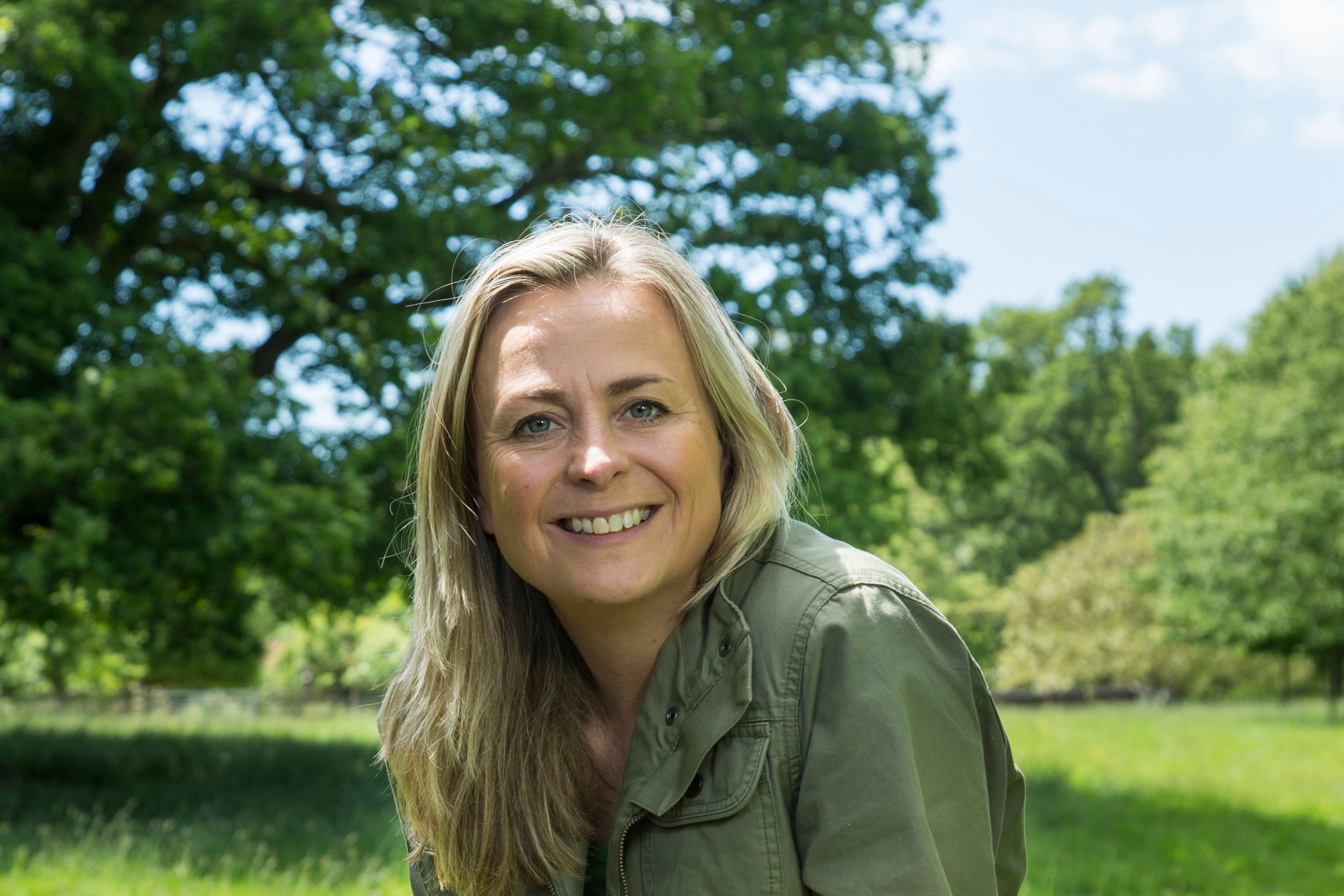This photograph features a smiling Caucasian woman with striking blue eyes and long, layered blonde hair that contrasts with her much darker eyebrows, suggesting that her hair may be dyed or that she naturally has dark blonde eyebrows. She is outdoors, sitting in a sunlit field of grass, with the light casting gentle shadows across her face and torso. She is facing the viewer and slightly leaning forward in a relaxed pose. She's dressed in an olive green jacket that suggests a military, safari, or field style, complete with a breast pocket.

In the slightly blurry background, you can see a tranquil outdoor setting with many green trees and a blue sky adorned with a few wispy white clouds in the top right corner. There's a noticeable larger tree on the left-hand side of the image, with more open sky visible on the right. This setting, combined with her attire, evokes the image of an adventurer, scientist, or anthropologist at work in the field. The natural, makeup-free appearance of the woman enhances the authentic and picturesque quality of this likely spring or summer scene.